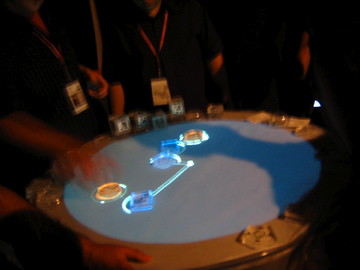The photograph captures a dark, blurry scene centered around a high-tech, light-interactable game table with a distinctive round design. The table features a brown outer edge and a light blue circular screen at the center, equipped with multiple clear plastic pucks illuminated by distinct LED lights, including two orange pucks and three blue pucks. Surrounding the table are several people, either standing or possibly sitting, as they interact with the pucks by touching or pointing. Many of the individuals wear lanyards with badges or name tags, hinting at a formal or organized event. The image’s blurriness and poor lighting obscure facial details and give everything a fuzzy appearance, creating an almost glowing effect that makes it difficult to discern finer details like a hand in motion or other potential objects on the table.